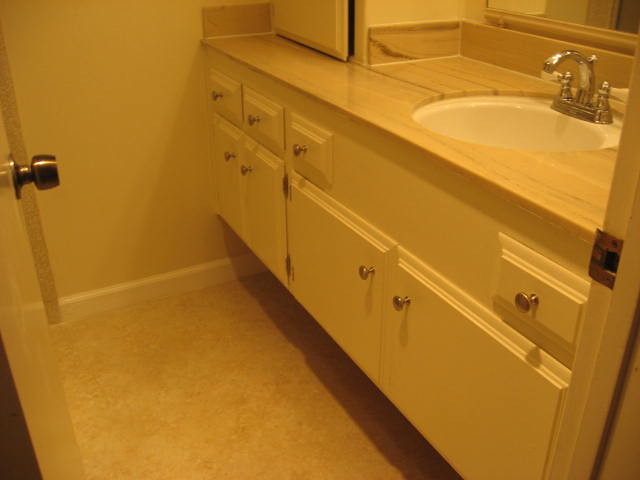This image captures the interior of a bathroom from a side view, showcasing various details. The bathroom door is open, providing a glimpse into the space. Dominating the scene is a white sink set into a light brown, wood-finished countertop. The sink itself is pristine white, complete with a central basin and a silver faucet mounted on the countertop.

Above the sink, a mirror is mounted on the wall, perfectly aligned with the faucet beneath it. The vanity features multiple storage options with its white cabinetry: four drawers—three aligned on one side and one standalone—and cupboards with either small or spacious shelves, ideal for various storage needs. The entire area is well-tiled, contributing to the overall clean and organized appearance of the bathroom.